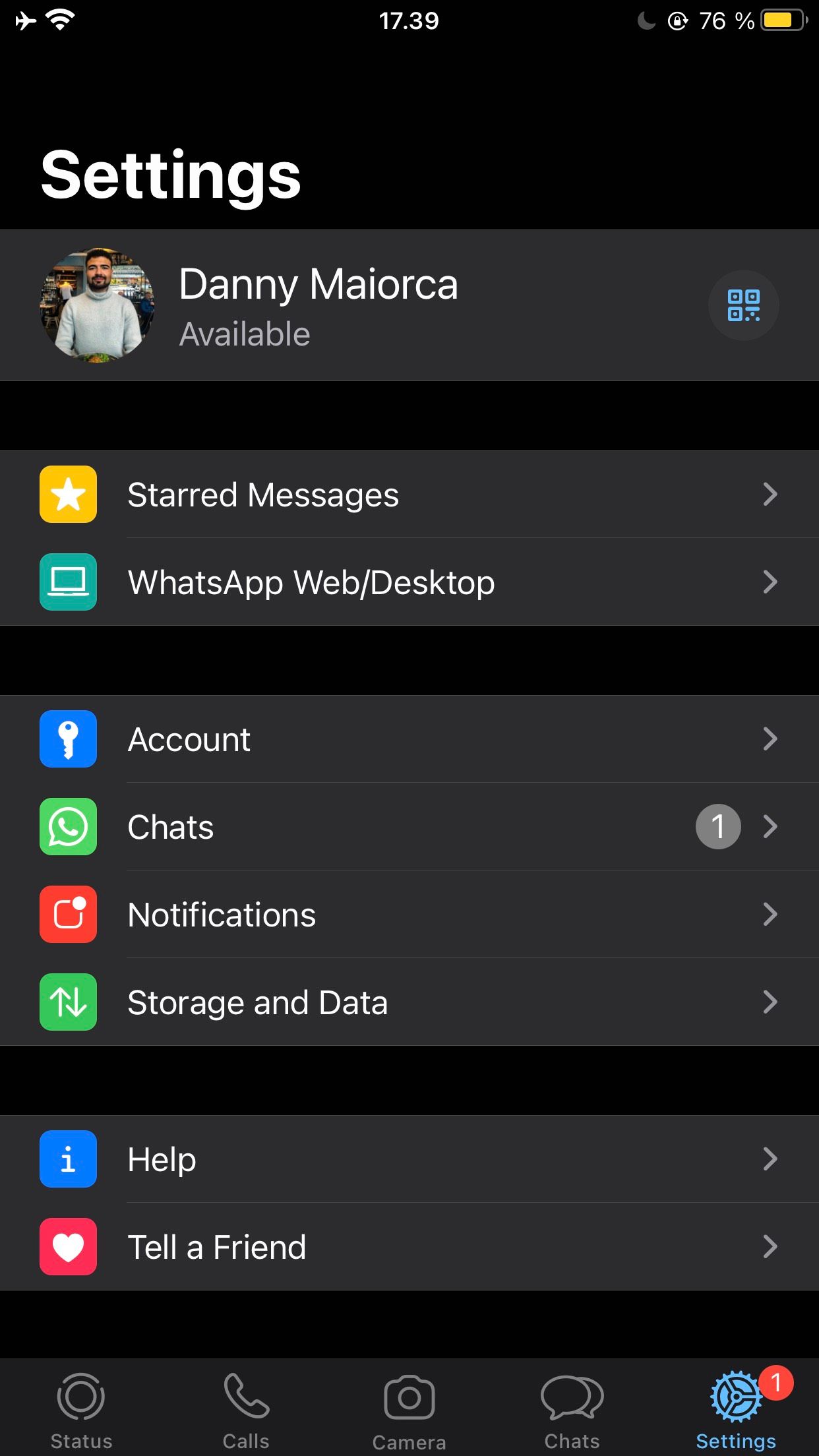This is a cell phone screenshot capturing the settings page of an app, presumably WhatsApp, displayed on a user's device. At the top left corner, just beneath the status bar showing cell phone signal strength, WiFi, battery life, and the time (17:39 or 5:39 PM), the page is titled "Settings."

Below the title, there is a user section featuring the name "Danny Maiorca." To the left of this name is a round profile picture showing a man with black hair and a beard, wearing a white sweatshirt, and facing directly towards the camera. Underneath the name, in smaller fonts, is the status "Available."

Next, there is a section titled "Starred Messages" followed by "WhatsApp Web/Desktop," both accompanied by respective icons to their left.

The subsequent section includes four setting options:
1. **Account** - Represented by a key icon.
2. **Chats** - Indicated by a speech bubble icon.
3. **Notifications** - Marked with a bell icon.
4. **Storage and Data** - Signified by a storage icon.

At the bottom of the page lies the final section containing:
1. **Help** - Accompanied by a question mark icon.
2. **Tell a Friend** - Denoted by a speech bubble icon with an arrow.

The detailed layout, inclusive of user details, categorized settings, and an organized icon-based menu, presents a comprehensive visual account of the user’s settings interface.